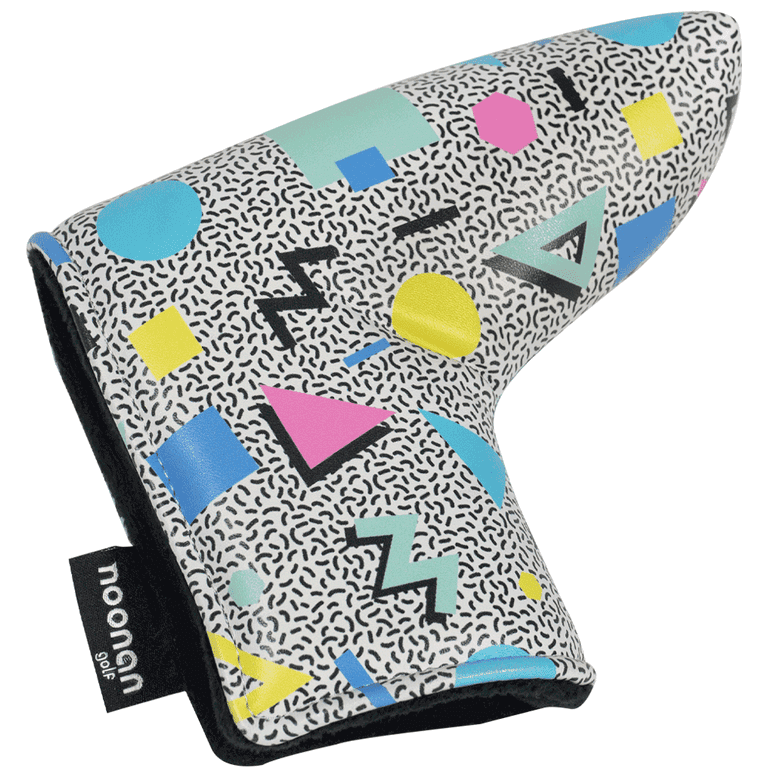This image prominently features a club head protector for a golf club. The protector boasts a distinctive retro aesthetic, reminiscent of late 80s or early 90s design. It is shaped somewhat like an inverted boot, with an opening designed to slide over and encase the head of a golf club. The exterior of the protector is adorned with a white background, speckled with small, black, sprinkle-like patterns that evoke the appearance of cake decorations or thin jelly beans. Complementing this pattern, the protector also displays an array of vibrant geometric shapes, including pink triangles, blue and yellow squares, and circles, scattered in a seemingly random fashion.

A black tag attached to the protector clearly reads "Noonan Golf," confirming its use as a golf accessory. The interior fabric of the protector is black, which provides a sleek contrast to its vivid exterior. The combination of polystyrene or a soft foam core wrapped in synthetic material ensures both durability and protection for the golf club. Overall, the design elements and construction details underscore its intended function while offering a playful nod to retro graphic design trends.